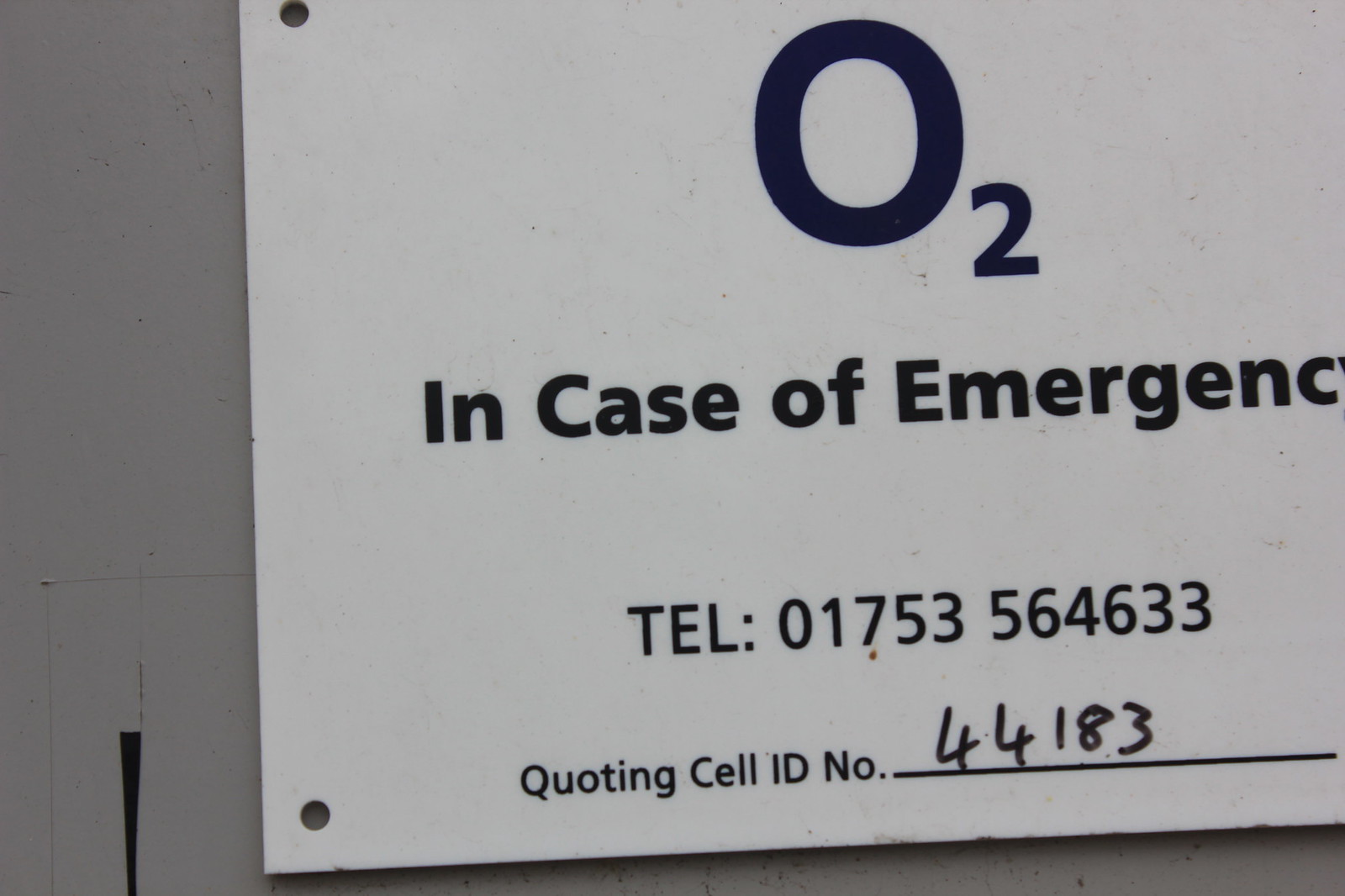This detailed photograph features a close-up of a white emergency sign attached to a wall, which appears either white or gray. Notably, the sign has two holes, one in each of the upper left and bottom left corners, suggesting it is fastened securely. Dominating the signage in large black text is "O2," with the number 2 positioned slightly lower. Directly beneath this, in smaller black text, the sign states: "In case of emergency." Below this instruction, it reads: "TEL: 01750564633," though one interpretation notes the number could alternatively be "01753-564-633." Further down, another line of text instructs, "quoting cell ID number," followed by an underlined area where the number "44183" is handwritten in black marker. This entire arrangement sits against a white wall that exhibits red stains at its base.